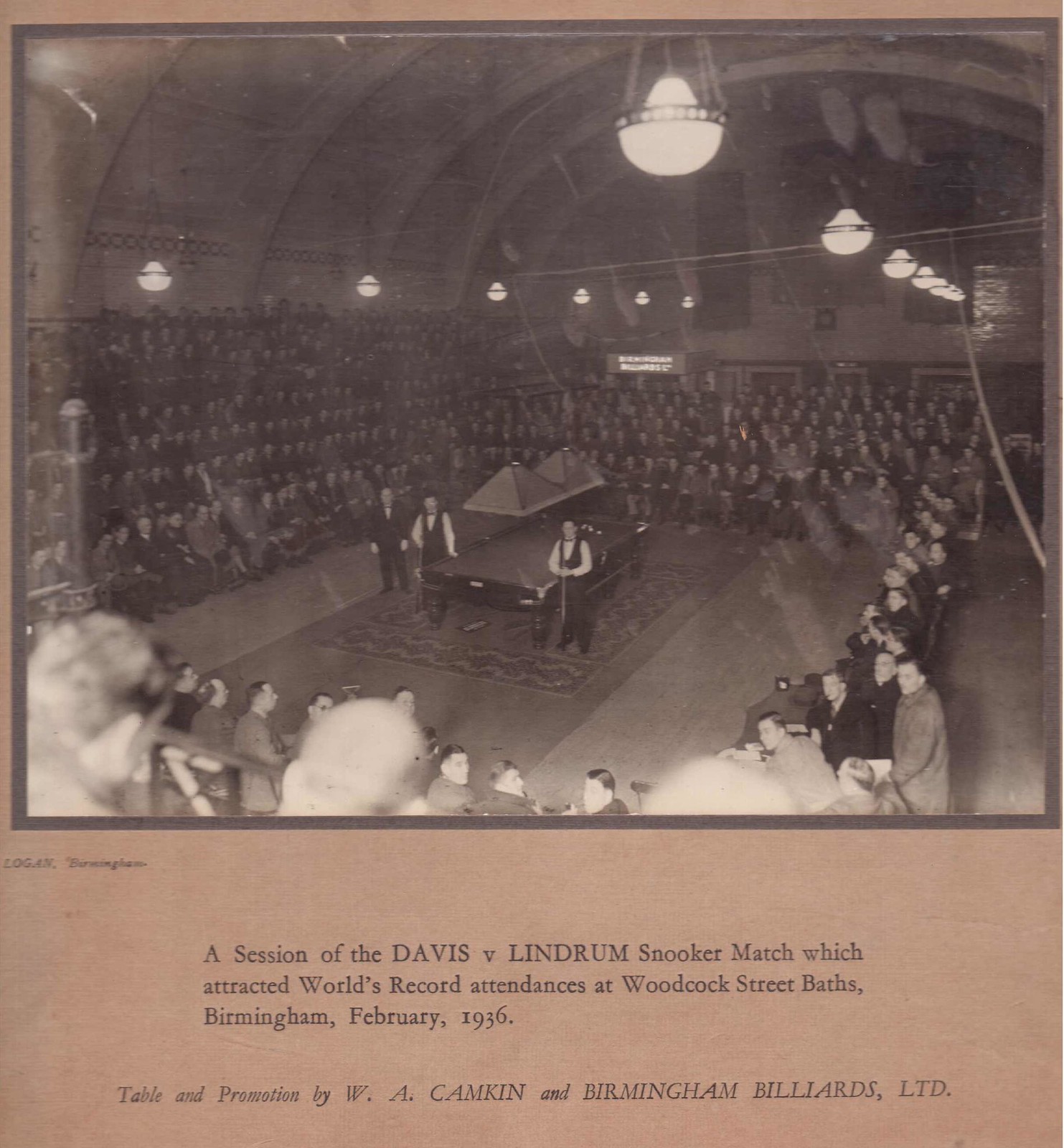The image is a black-and-white photograph set within a brownish or pinkish bordered poster. The photograph captures an indoor snooker match held at the Woodcock Street Baths in Birmingham, February 1936, during the Davis vs. Lindrum encounter, renowned for attracting a record-breaking audience. In the center, a well-lit snooker table rests on a rug, with two players dressed in black vests, white shirts, and black pants, holding snooker cues. Surrounding the table, a large, attentive crowd sits in various sections, including bleachers on the left, seats along the edges, and more individuals at floor level. The venue features a high, arched ceiling with additional light fixtures providing illumination. The promotional text below the image credits WA Campkin and Birmingham Billiards Ltd for the event.